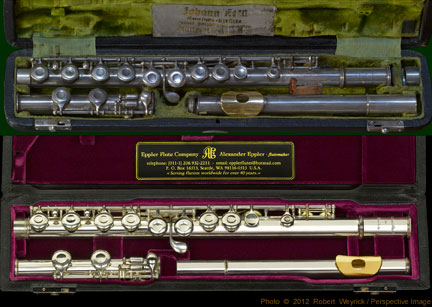The image is of two disassembled flutes displayed in their respective cases, which are positioned one behind the other. The photograph is slightly wider than it is tall, making it somewhat challenging to discern finer details. Each case holds a flute neatly split into sections. The upper case contains a newer, shinier flute with a silver body and a gold mouthpiece, laid out in two sections: the longer upper flute part and the combined lower third and two-third segments. The interior of this case is lined with a luxurious light green velvet.

The lower case houses a slightly older flute made of gold-colored metal, also featuring a gold mouthpiece. It, too, is divided similarly into a long upper segment and two smaller lower segments. The inside of this case is lined with rich red velvet. Both cases include small plaques with elegant gold writing, suggesting high-end promotional material for an upscale music store. The plaque in the red velvet case is more prominent and appears to be black with gold lettering, adding a touch of sophistication. The green velvet case includes a smaller, undecipherable cloth tag with gold letters.